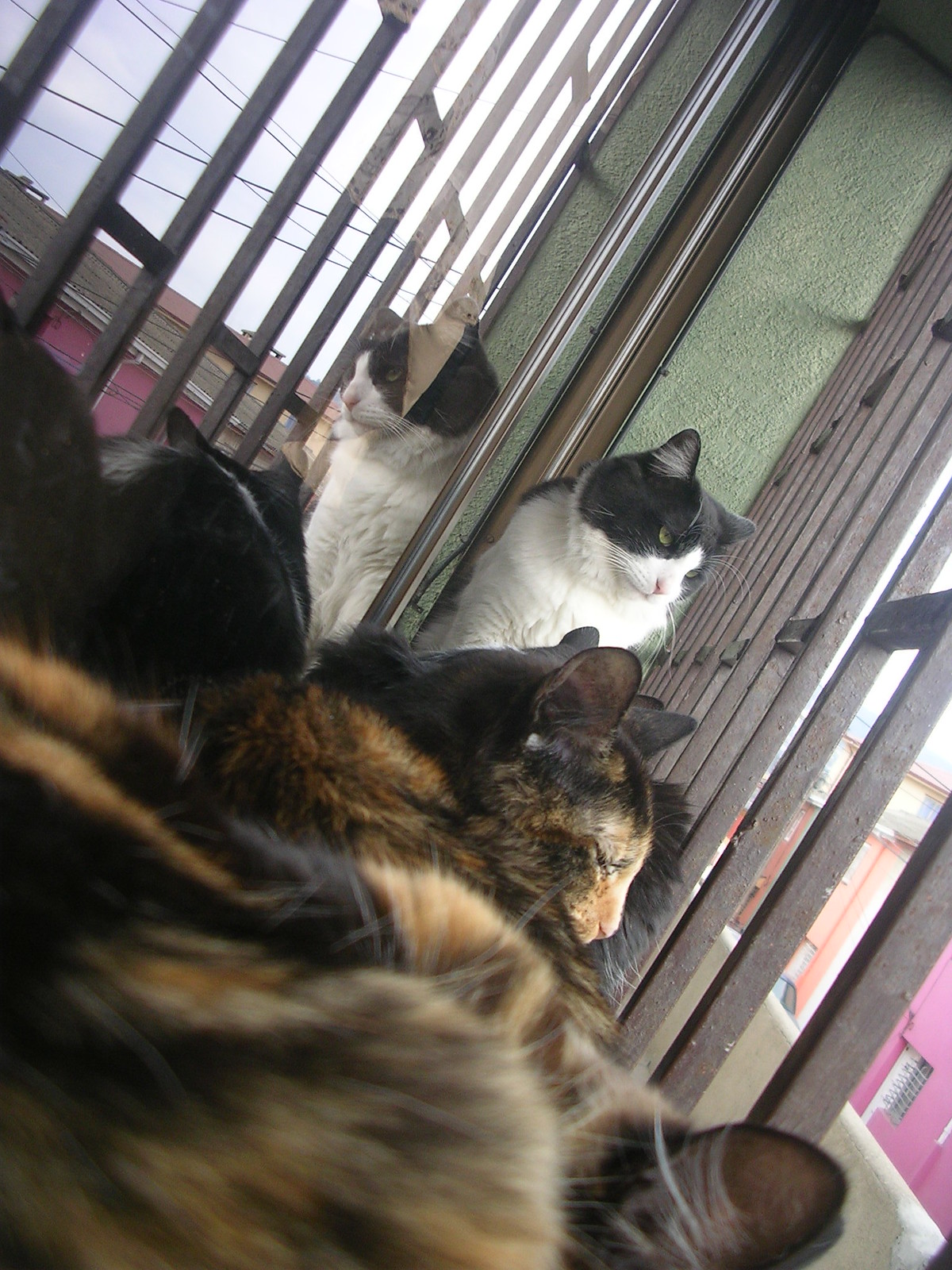In this detailed photograph, we observe a narrow windowsill where four cats are perched, all intently gazing out through a caged window. The first cat, nearest to us, exhibits a striking tiger pattern of brown and black fur. Next to it, there is a black and white cat, notable for its distinctive black face with a white mouth and the middle of the face, with white shoulders and legs. The third cat appears to be jet black. Lastly, there is a partially visible cat, suggested by its ears peeking out. The cats have medium-length fur, neither long nor short, and they are attentively viewing the vibrant street outside. Across the way, colorful buildings—lavender and orange—adorn the scene with their own caged windows, enhancing the photograph's depth. The image is illuminated by daylight, which is reflected both on the cats and the window, creating a serene yet lively atmosphere.